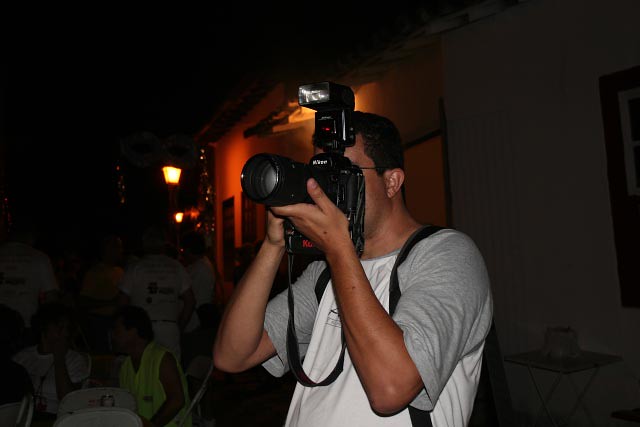This photo captures a man taking a photograph with a high-end, black camera equipped with a large lens and a flash. The man, who has short hair and wears glasses, holds the camera up to his face, obscuring it. He is dressed in a short-sleeve shirt that is predominantly white with gray sleeves, and a camera strap hangs around his neck. The setting is dark, suggesting nighttime, and the scene is outside in front of a house where a party appears to be taking place. The porch light and additional light on the left side illuminate the area just enough to reveal details like the presence of other people in the background. One notable detail is a woman in a sleeveless green shirt positioned to the left of the man's right elbow, seemingly looking at him. The dim lighting creates a soft ambience, and you can faintly see the off-white wall and small table behind the man, along with some darker, shadowed areas that are difficult to discern.